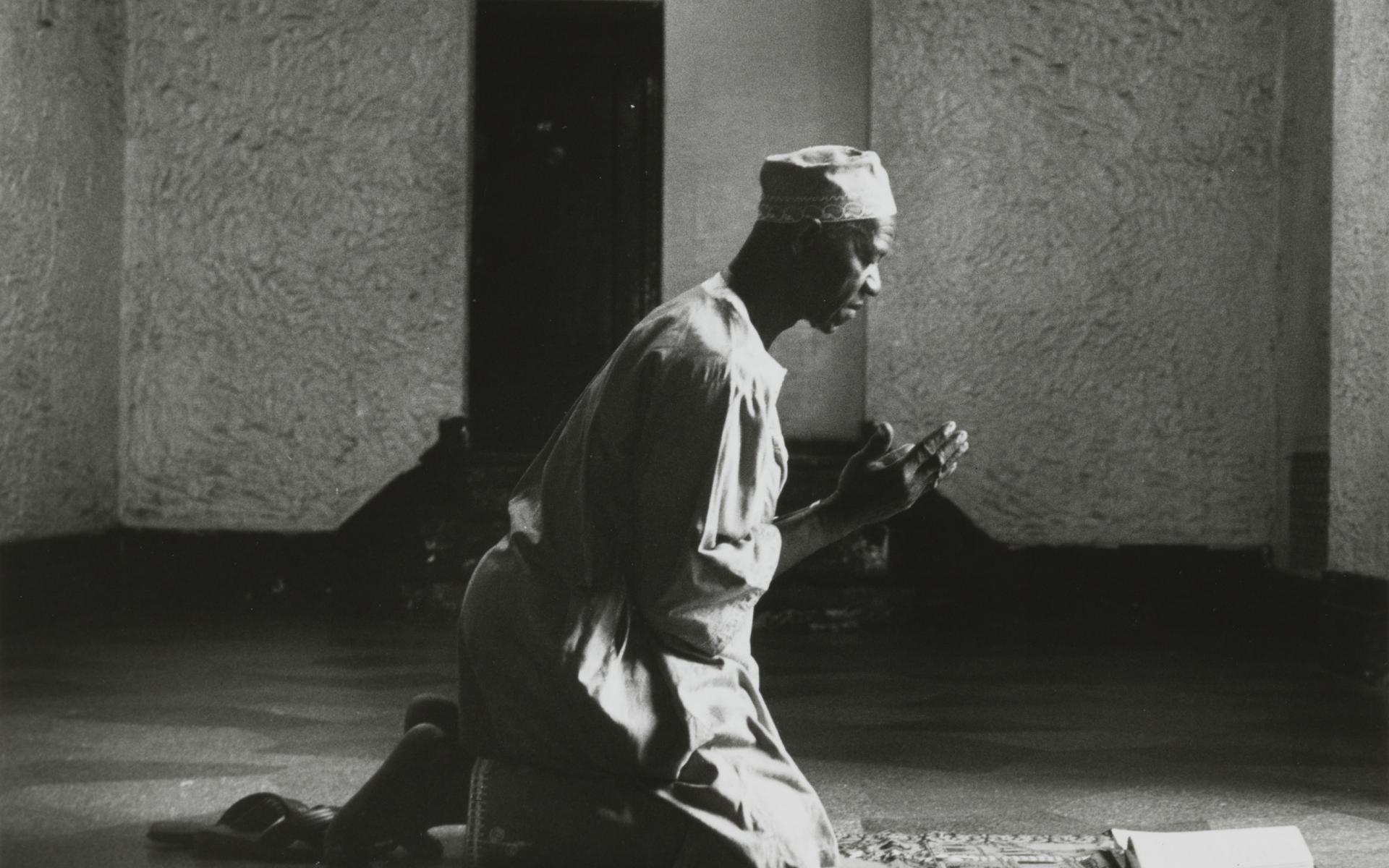The black and white vintage photograph captures a moment of deep prayer. The image depicts a dark-complexioned, middle-aged man, likely of Islamic faith, kneeling on a floral-patterned carpet inside a spacious, plain room with whitish gray walls and what appears to be a dark door and adjacent stairs in the background. The man is oriented towards the right side of the frame, where light seems to be streaming in, perhaps from a window. He is dressed in a long robe and a plain, round cloth hat, without a brim. His eyes are closed as he holds his hands in a prayerful gesture, palms open and close to his chest. His sandals are neatly placed beside him, suggesting he is barefoot or in socks. The floor appears to be tiled in varying shades of gray. There is a collection of white pages or a book in front of him, adding a focal point to his devotion.